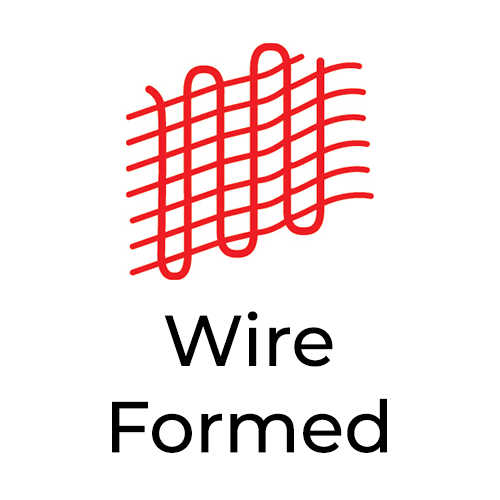The image features a white background with a centrally placed cartoon-like, computerized drawing in red. Dominating the top portion of the image are seven diagonal wavy lines that ascend from the lower left to the upper right. Intersecting these wavy lines is a series of vertical, looping lines that rise and fall in a continuous motion, reminiscent of a loop-de-loop or sheet music. This intricate design resembles a uniquely formed grid or a maze of tightly wound strands, not unlike the shape and form of a paper clip. Beneath this intricate assembly, in large black letters, are the words "wire formed." The entire composition is centered, with the text aligned directly below the red graphic elements.